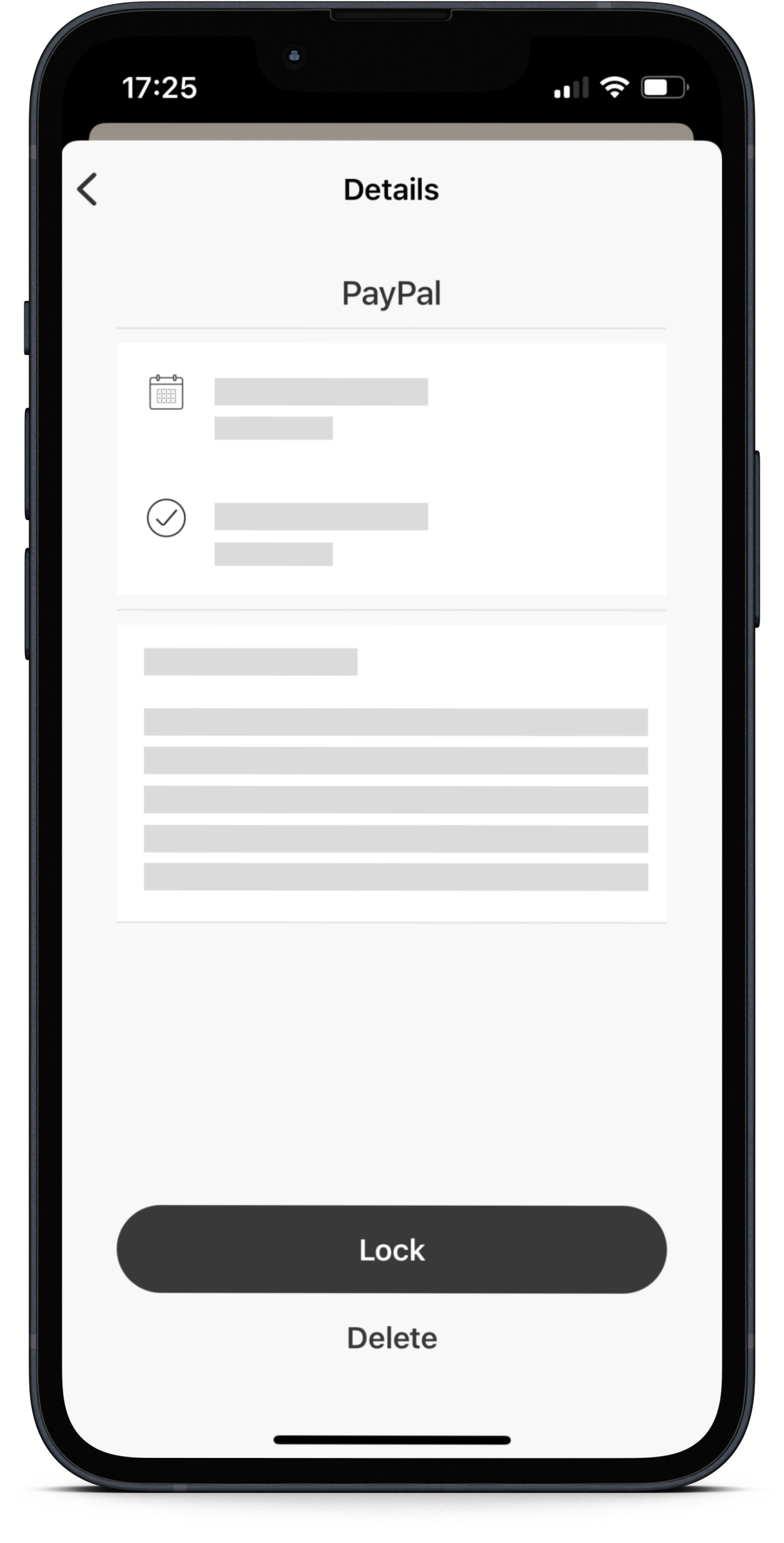This image showcases a smartphone, highlighting both its physical and on-screen elements. The phone, encased in a black border, displays the time in the top-left corner as "17:25" in white text. Adjacent to the time, two signal bars indicate mobile reception, and the Wi-Fi icon shows an active connection. The battery icon, positioned further right, is just above 50%, though it lacks a numeric percentage indicator.

Interestingly, the phone screen features a poorly Photoshopped layer over it, which does not align perfectly with the phone's display. The background of this overlay is stark white, revealing the phone's screen behind it at the top.

On the top-left corner of the Photoshopped section, there are two lines forming a left-pointing arrow. Centered at the very top of this section, the word "Details" is prominently displayed. Directly underneath, the text "PayPal" is written with a mix of capitalization: capital "P," lowercase "a," capital "Y," lowercase "P," and so forth.

Below this "PayPal" text, a calendar icon appears on the left, next to which is a gray bar. Directly under this, a shorter gray bar is half the length of the one above it. Following this, a circle encompassing a check mark is shown with another gray bar beside it, and below that, yet another shorter gray bar.

Further down the layout, there is a slightly extended gray bar, followed by a series of five fully extended gray bars. At the bottom of this arrangement, two symbols are visible: a lock and a delete icon.

The juxtaposition of the actual phone elements with the misaligned Photoshop overlay creates a cluttered and confusing image.